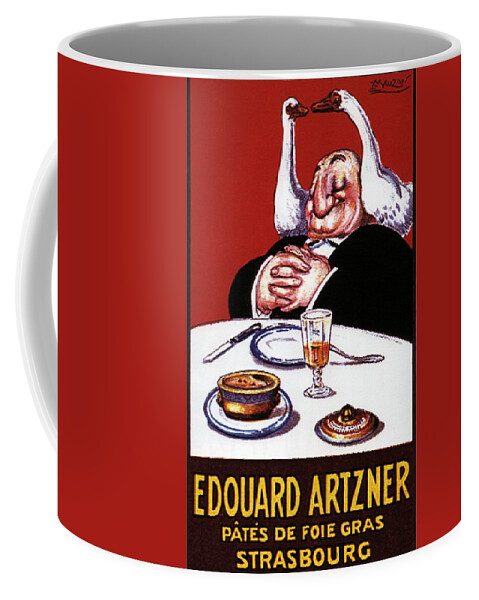This detailed close-up shot features a red mug with a white interior and handle. The central design is framed by two black lines, showcasing an illustration of an overweight man with a slightly disfigured face, dressed in a black suit. The man's hands, notably large compared to his body, rest on his belly. Poised on his shoulders are two white birds—resembling ducks or swans—with their beaks almost touching in a mirrored position. The man is seated at a round table set with a white tablecloth. Before him lies an empty plate accompanied by a knife, a glass half-filled with amber liquid, and another plate holding a jar of something brown, likely pâté or foie gras, with its lid beside it. Below this image, a black banner with gold-yellow capital letters reads "Edouard Artner, Pâté de Foie Gras, Strasbourg."